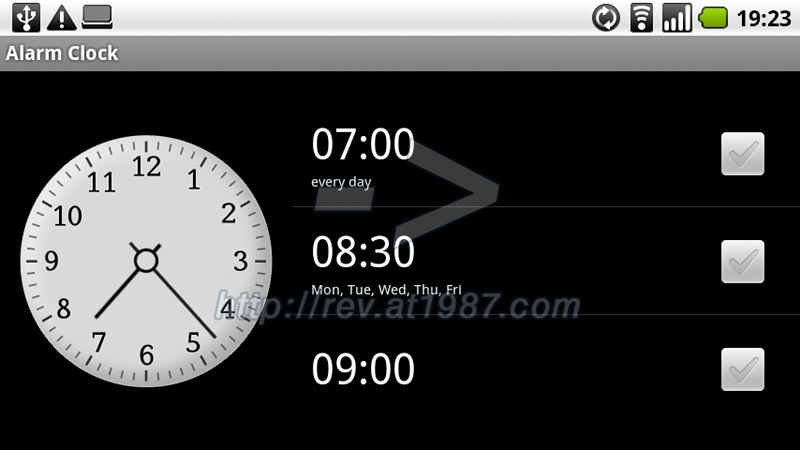This detailed caption is for a screenshot taken from a mobile phone in landscape orientation. In the top left corner, the text "Alarm Clock" is visible. On the left side of the screen, a digital clock face displays the time "7:23." The screenshot shows a list of alarms set on the device: a recurring alarm set for 7:00 AM every day, another recurring alarm set for 8:30 AM from Monday to Friday, and a final alarm set for 9:00 AM with no specified recurrence. A watermark partially obscured by the white clock face reads "P: LLREV.AT1987. com," with some letters difficult to discern.